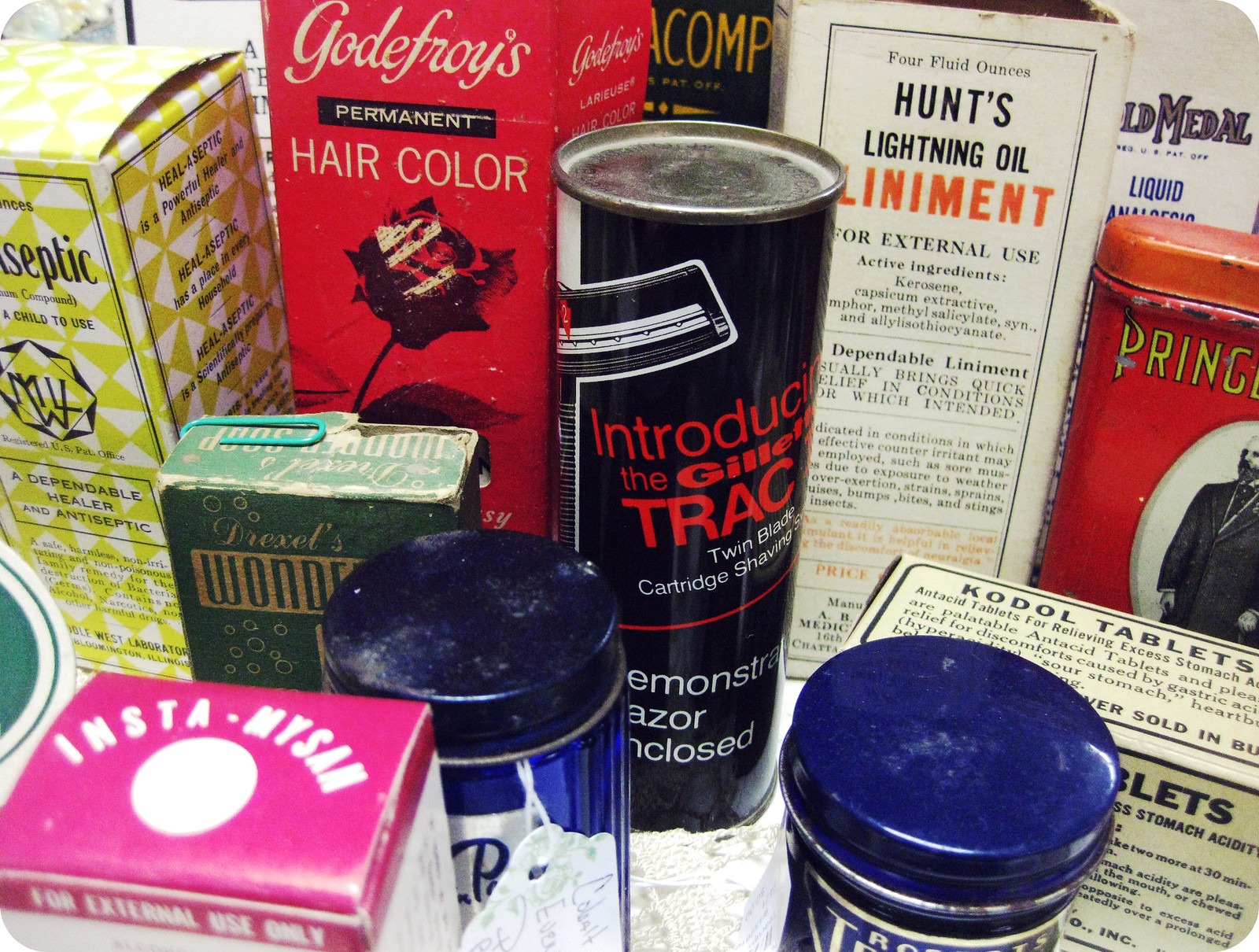This detailed photograph showcases an assortment of vintage toiletry products, each item seemingly a blast from the past. Starting from the left, there's a yellow and white box prominently labeled "Antiseptic, a Dependable Healer." Next to it stands a red rectangular carton featuring a black rose, titled "Godfrey's Permanent Hair Color." In front of this box lies a green container, "Drexel's Wonder Soap," secured with a green paperclip on top. Moving further right, there's a notable black tin can advertising "Introducing the DELECTRAC Twin Cartridge Shaving" with the phrase "Razor Enclosed" at the bottom. Furthermore, among these items, other vintage casings are visible, including a white box marked "Hunt's Lightning Oil Liniment for External Use" and a container of "Kodol Tablets." Also spotted on the right is a familiar "Prince Albert Can." This eclectic collection sits atop a shelf, each item tagged with notes, likely indicating they are on sale.